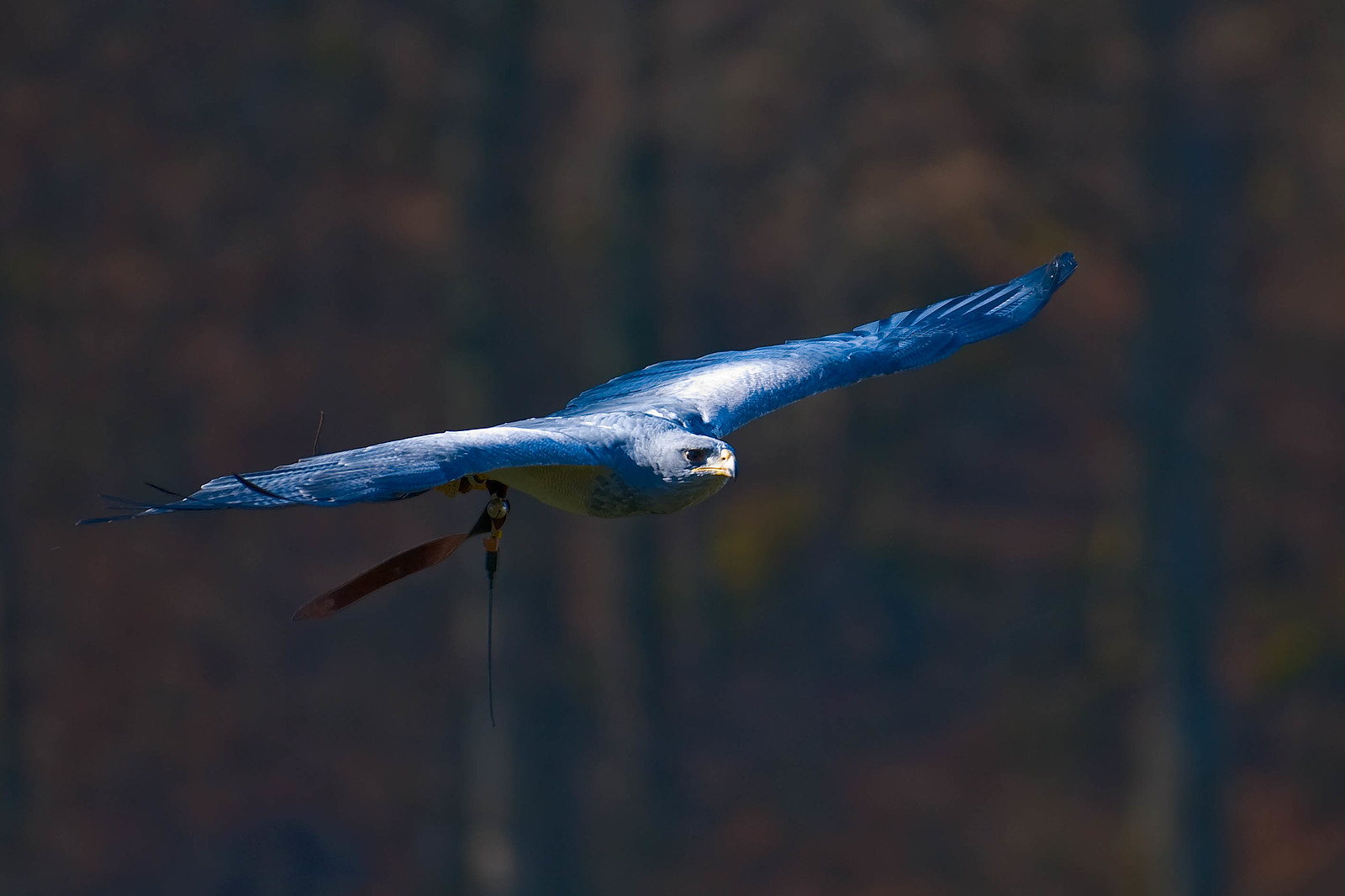This detailed nature photo captures a strikingly vibrant blue bird, possibly a falcon or another bird of prey, gliding effortlessly through the air with its wings fully outstretched. The bird's vivid blue feathers shimmer in the light, highlighted by subtle white and yellow accents. Its large, sharp eyes and a yellow beak add to its imposing appearance. The bird appears to be carrying something with one of its talons—a feather-like end of a fishing line or perhaps a leather strap with a silver ball and string, possibly indicating it is a messenger bird or has been tagged by a nature agency for conservation purposes. The background is artistically out of focus, creating a purplish-brown bokeh effect that makes the bird stand out even more dramatically against the blurred hints of a forest setting.